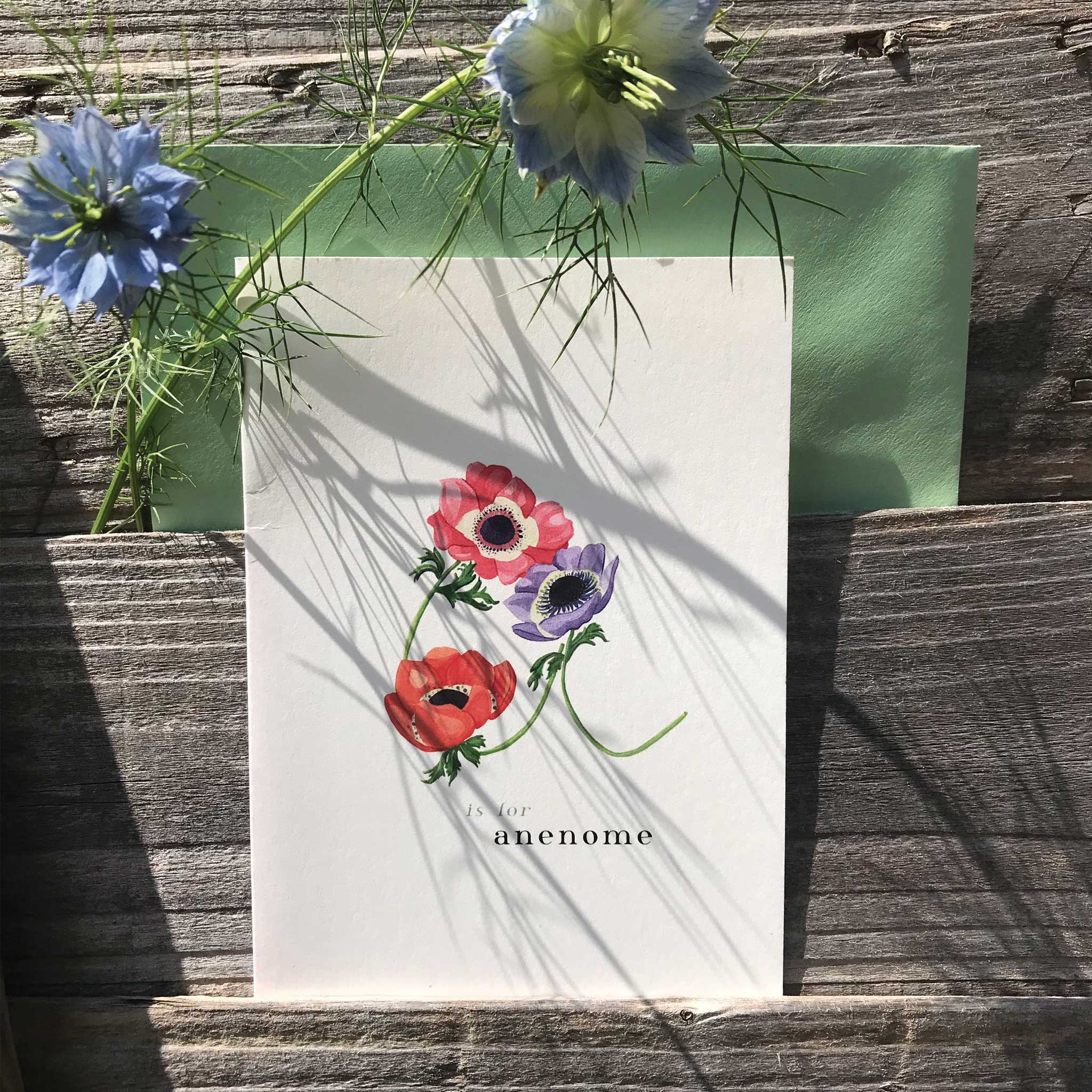This photograph showcases a minimalistic white card featuring three flowers—pink, red, and lavender—arranged to form the letter "A." The stems of the flowers, which are green in color, creatively shape the letter as part of the text, "A is for anemone." The card is positioned against a backdrop of three wooden panels bathed in sunlight. A green envelope sits behind the card, adding an additional layer to the composition. Above the card, there are real blue flowers with a greenish tint in the middle of their petals, contributing to the natural and chaotic feel with their shadows cast on the card. The bright sunlight illuminates the scene, creating distinct shadows of the flowers and leaves on the white surface, blending real and graphic elements in an intriguing manner.